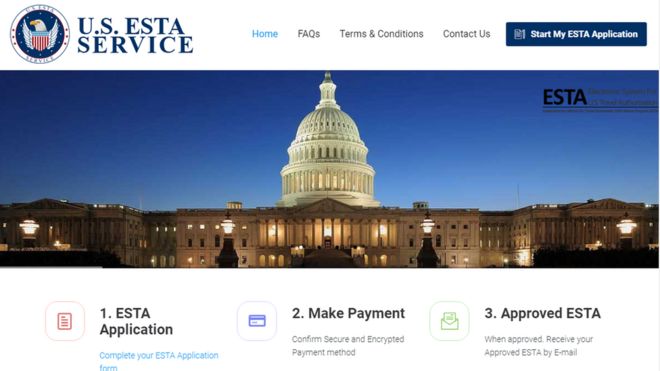This image features an official webpage from a federal government website, specifically the U.S. ESTA (Electronic System for Travel Authorization) Service. At the top of the page, there is a seal with an eagle emblem, although its design appears somewhat lackluster, depicting an eagle with clipped wings. 

The main title "U.S. ESTA Service" is displayed prominently in blue. Navigation options are listed horizontally across the top of the page and include "Home," "FAQs," "Terms and Conditions," "Contact Us," and "Start My ESTA Application," the last of which is a clickable blue tab.

Below the navigation bar, a large photograph of the U.S. Capitol building at night spans the width of the page. In the upper right-hand corner of this image, the word "ESTA" is printed in black text—an unfortunate color choice that makes it difficult to read against the dark background.

At the bottom section of the page, there are three interactive icons, each with a corresponding logo: a red icon for "ESTA Application," a blue icon for "Make a Payment," and a green icon for "Approved ESTA." These icons offer users the ability to complete an ESTA application, confirm payment through a secure and encrypted method, and receive approval notifications via email.

Note: The Electronic System for Travel Authorization (ESTA) is a U.S. government program that determines the eligibility of visitors to travel to the United States under the Visa Waiver Program (VWP).